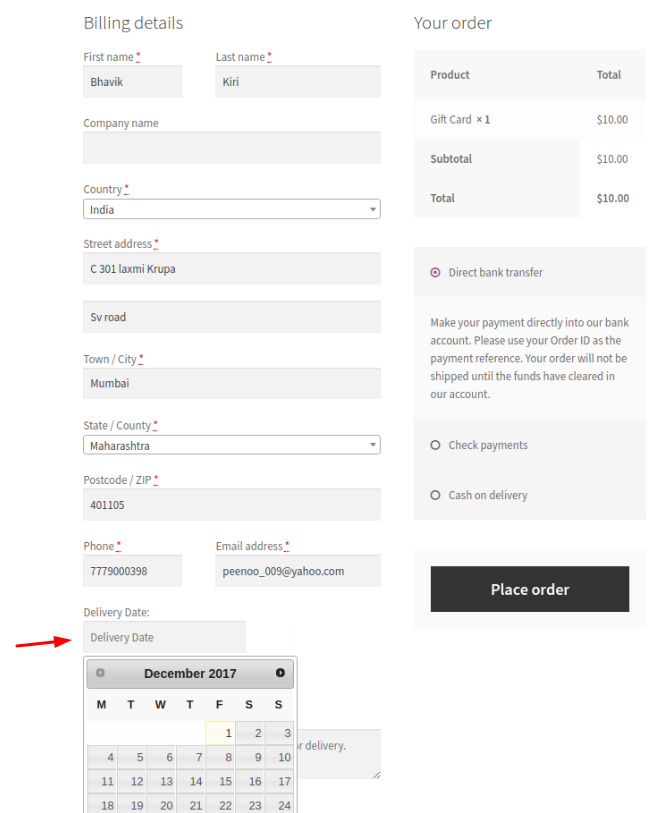This image is a detailed screenshot of the order page on a website. The background is predominantly white with elements like text boxes and buttons in shades of gray and black.

### Right Section: Your Order
- **Header:**
  - In gray font, "Your Order" is prominently displayed.
- **Order Details:**
  - Below the header, gray rectangular boxes outline the summary of the order.
  - **Product**: Listed as “Gift Card x 1”
  - **Total**: Each of these line items—Product, Subtotal, and Total—have a corresponding amount of $10 indicated.
- **Payment Method:**
  - "Direct Bank Transfer" is the selected payment option.
  - The instructions below inform the user: "Make your payment directly into our bank account. Please use your order ID as the payment reference. Your order will not be shipped until the funds have cleared in our account."
  - Alternative payment options such as "Check Payments" and "Cash on Delivery" are also listed below.
- **Action Button:**
  - A clickable black rectangle with white font is located at the bottom. It reads "Place Order."

### Left Section: Billing Details
- **Header:**
  - The section begins with "Billing Details" in gray font.
- **Form Fields:**
  - **First Name**: Filled in as "Bhavik"
  - **Last Name**: Filled in as "Kiri"
  - **Company Name**: Left blank
  - **Country**: Selected as India
  - **Street Address**: "C 301 Lakshmi Krupa, SV Road"
  - **Town/City**: "Mumbai"
  - **State**: "Maharashtra"
  - **Postcode/Zip**: "401 105"

This comprehensive description provides a clear visual of the page layout and the user inputs, facilitating an understanding of the order process and the necessary details for completing a transaction.